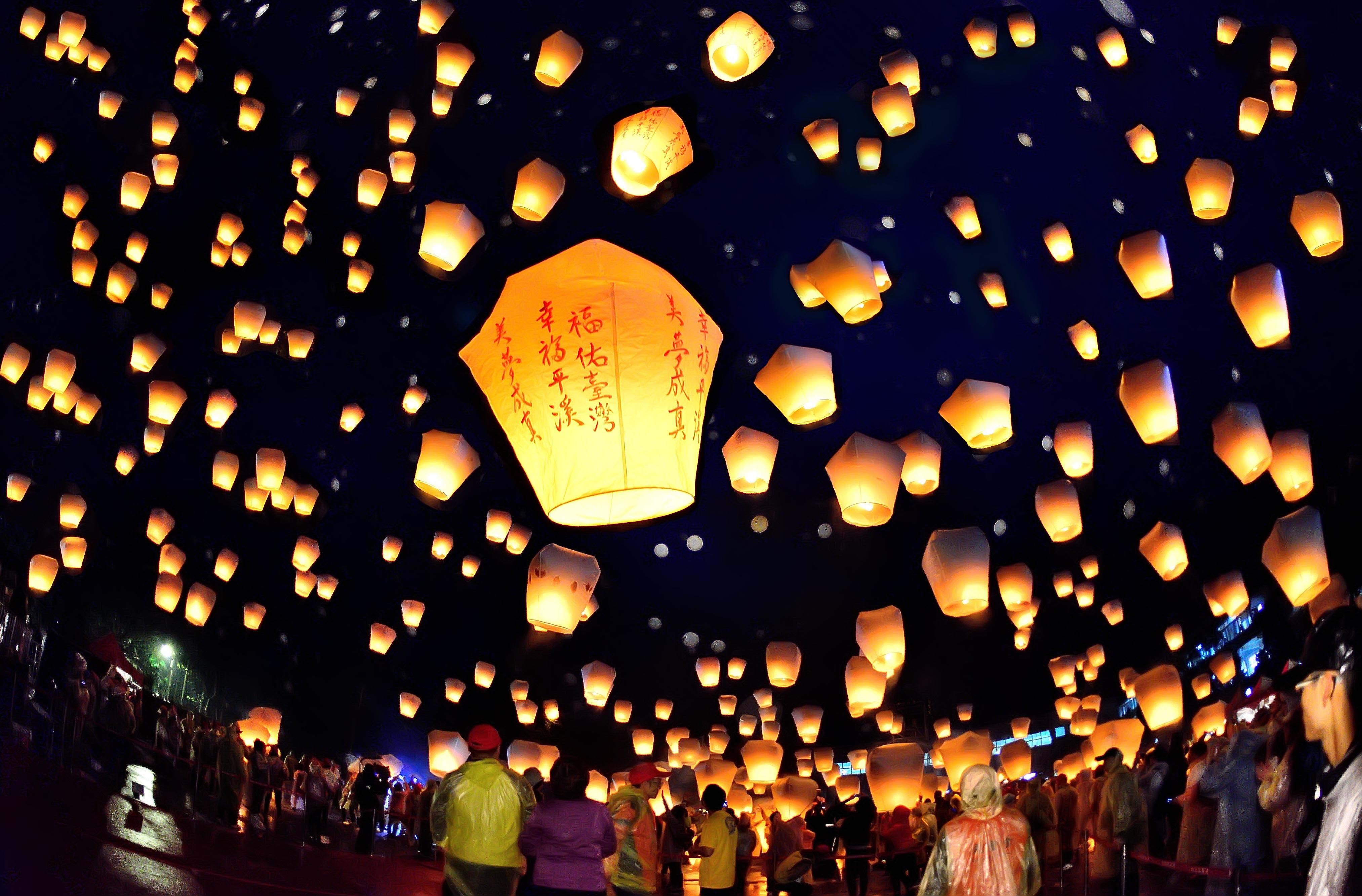This photograph captures a mesmerizing moment at an Asian festival or ceremony where hundreds of illuminated paper lanterns are released into the night sky. The pitch-black background dramatically highlights the glowing lanterns of various sizes, creating a captivating visual effect as they ascend. At the center of the image, slightly to the left, one prominent lantern displays Asian writing, the characters clearly visible against its light. The crowd of over 200 people at the bottom of the image is mostly turned away from the camera, gazing upwards in awe. Many are adorned in translucent raincoats, suggesting a damp evening. Notably, on the left side of the image, a couple stands out, one wearing a purple jacket and the other a yellow one, both covered with clear raincoats. The crowd is arranged in a circular formation, possibly due to the wide-angle lens used, adding to the sense of community and shared experience at this enchanting event.